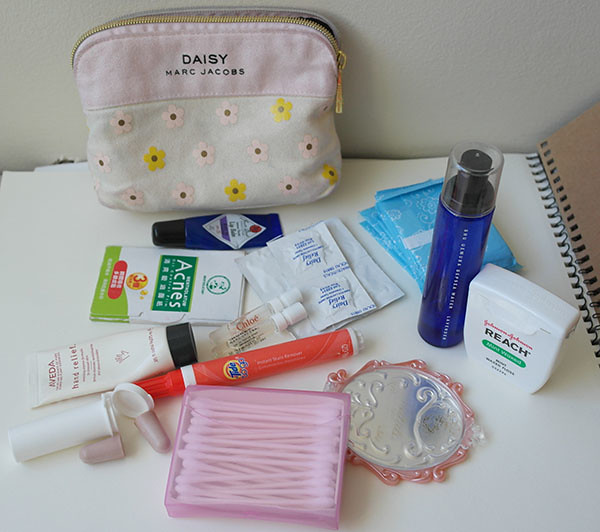The image portrays a white background, which is the open pages of a sketchbook with a spiral-style wire spine located on the right. The cover of the sketchbook is flipped open, revealing its plain brown cardboard interior. Positioned on the sketchbook’s blank pages, there is a small makeup bag prominently displaying the label "Daisy Marc Jacobs." The makeup bag features a gold-colored zipper, a pink fabric upper section, and a lower section adorned with a white fabric decorated with pink and yellow flowers.

Accompanying the makeup bag, there is a blue tube of cream with a black cap. Nearby, a small rectangular piece of cardboard is printed with the word "Acnes." Another cream tube is present, though further specifics aren't mentioned. Additional items include a small white plastic capsule with earplugs inside and a small pink container holding Q-tips. A Tide-To-Go pen, a container of dental floss, and a small mirror are also visible, completing the array of personal grooming and hygiene items laid out on the sketchbook background.